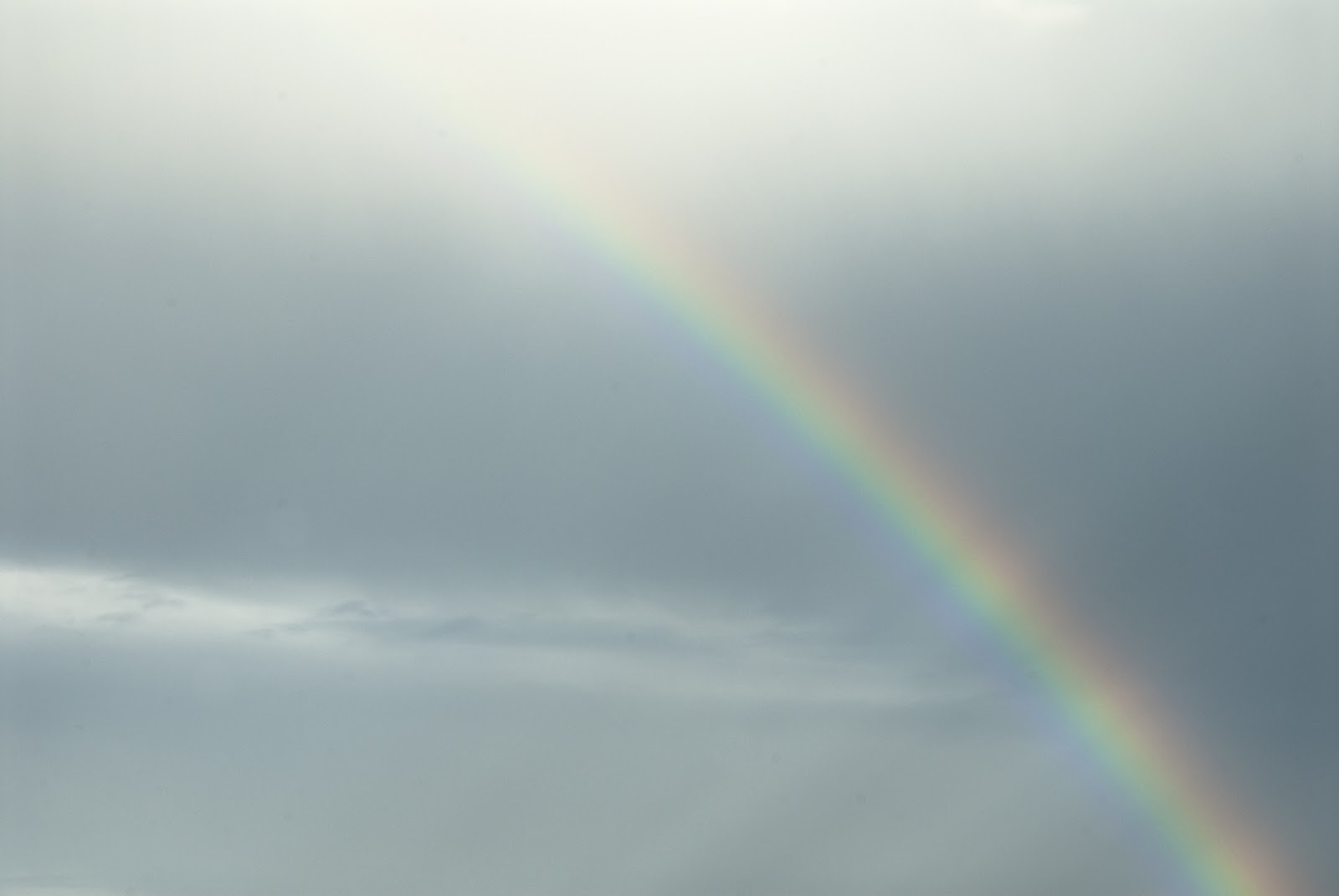In this image, a vibrant rainbow arcs across a heavily cloudy sky, stretching from the upper left to the lower right. The backdrop is primarily desaturated and murky, featuring black rain clouds interspersed with lighter gray and white clouds. The sky itself has a pale, greenish haze, possibly from recent rain, adding to the overall gloomy atmosphere. Despite this, the rainbow stands out vividly, showcasing a spectrum of colors: blue at the base, transitioning through green, yellow, and red, ultimately to purple at the top. There's a noticeable bright white light at the top of the image, likely from the sun breaking through the clouds, giving the scene a hazy, post-rain ambiance. The contrast between the rainbow's brilliant colors and the drab surroundings makes the rainbow the focal point, its colors sharply outlined yet slightly translucent.